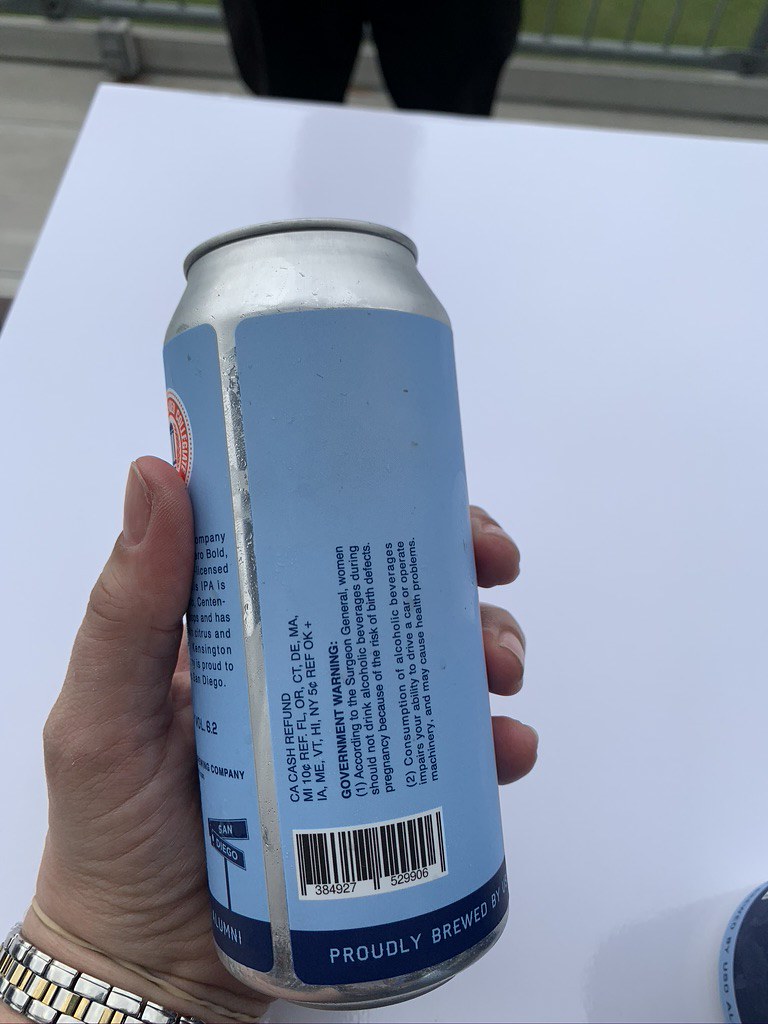In the image, a detailed scene unfolds: a wooden walkway barely noticeable in the background, suggesting an outdoor setting. On the left side, a person's fair-complexioned hand, adorned with a black, gold, and silver wristwatch, holds an aluminum can. The can has a silver top with a light blue label featuring a dark blue strip along the bottom, displaying a government warning, a barcode, and California cash refund text. A partially visible white tabletop is present, with a figure standing behind it, their legs cloaked in black pants and glimpses of a metal fence in the distance. The light captures the intricate details of the can and the subtle elements of the scene, providing a tapestry of textures and colors.